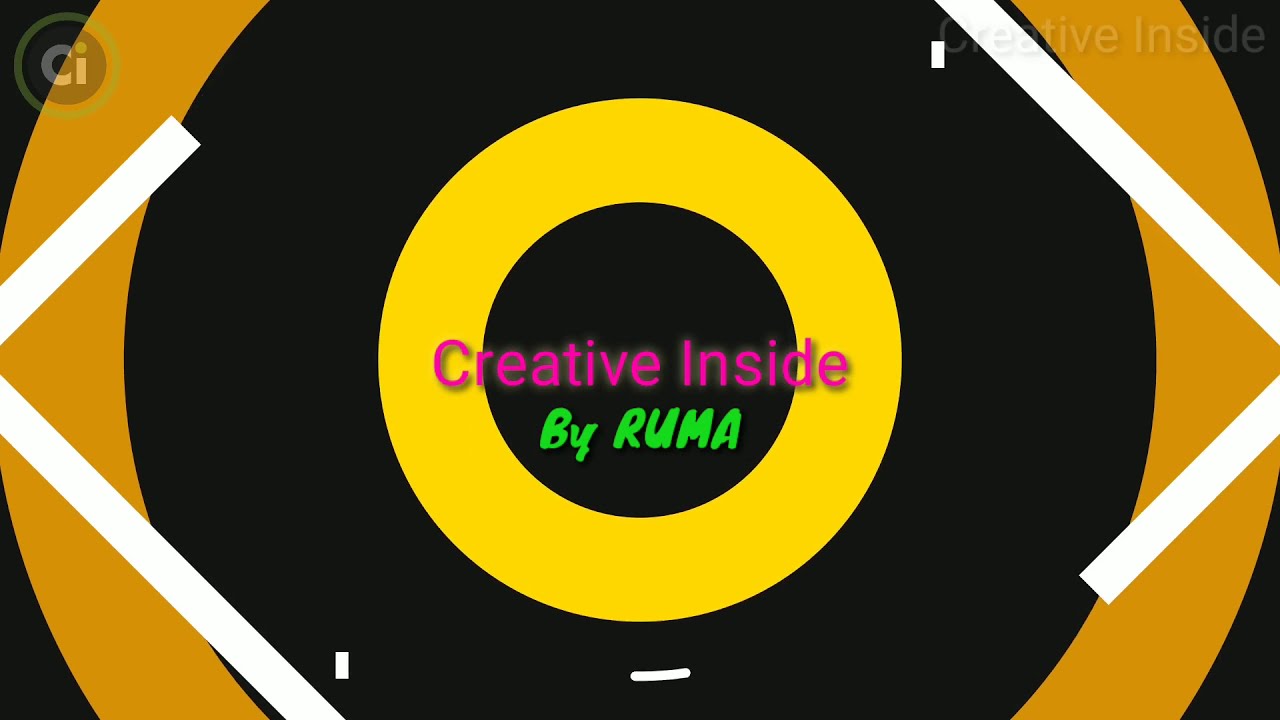This digital image prominently features a series of concentric circles filled with alternating black and yellow colors, reminiscent of a vinyl record. Starting from the innermost circle, the order is as follows: black, light yellow, black, dark yellow (sometimes described as orange), and finally a thicker black ring that reaches the outer edges of the image. The center of the design contains text that reads “Creative Inside” in pink sans-serif font, with “by Ruma” in green, handwritten-style font beneath it. In the top left corner, there is a circular logo with the initials “CI,” and in the top right corner, there is a watermark that also reads “Creative Inside.” The overall appearance of the design, along with its detailed text and complementary elements, creates an engaging, retro aesthetic.